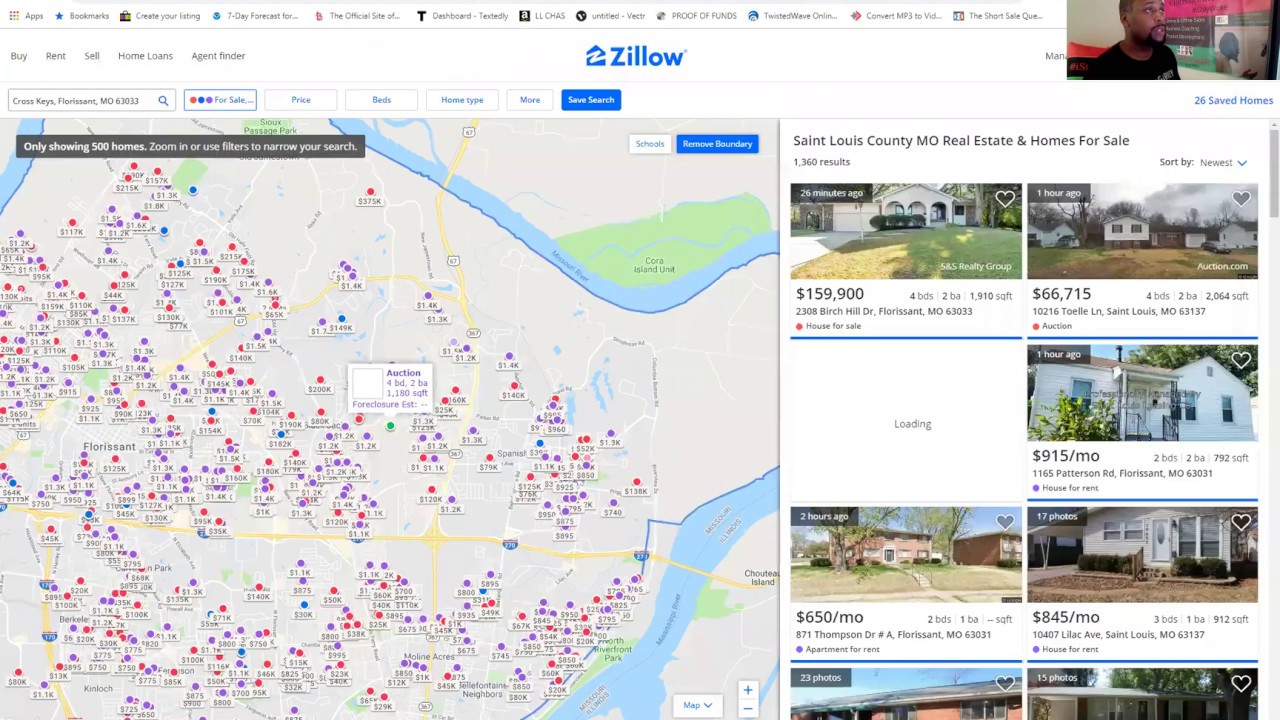**Descriptive Caption:** 

A Google Map view from Zillow showcasing real estate and homes for sale in St. Louis County, MO, is displayed with a variety of colored dots marking different properties. The map is dotted with purple, red, blue, and a few green markers, indicating different types of listings. The map is currently set to show a maximum brightness of 500 lumens.

Highlighted listings include:
- A house posted 26 minutes ago featuring a vibrant green lawn and a facade with three archways, listed at $159,000.
- A mobile home listed an hour ago priced at $66,000, with a placeholder image displaying "Loading."
- A small white house with a porch, listed at $9.15 per month.
- A brown apartment-style building with a rent price of $6.50 per month.
- A house with a covered carport, featuring two tall windows flanking the door and two shorter windows on the opposite side, listed at $8.45 per month.

Additionally, a small video overlay appears in the top right corner of the screen, showing a man seated in a room with a black and red sign behind him. He is wearing a black t-shirt. Various options like "Zoom in," "Save," "Remove Boundary," and "Sort By Newest" are visible on the map interface.